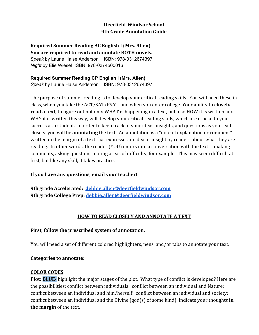The webpage features a minimalist design with a white background and black text written in an unreadable foreign language, resembling hieroglyphics. The content is organized into four large paragraphs, each separated by single lines. Mid-page, after the second full paragraph—which spans approximately ten lines—there are two blue hyperlinks. Directly below these hyperlinks is a centered and underlined line of text. Following this, there are two more single lines.

Further down, a bold line of text is present, which is succeeded by another line in all capital letters, albeit not bolded. Beneath this capitalized line, there is a sentence where the second word stands out as it is shaded in blue. This highlighted word is the only instance of this color usage on the page, and its meaning remains unclear. The content concludes with an additional four lines of text.